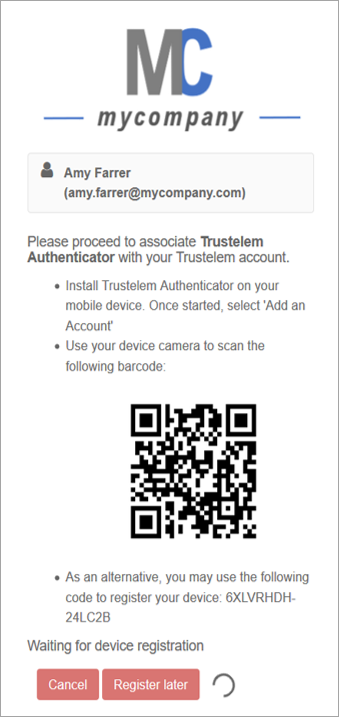**Detailed Image Caption:**

The image shows a screenshot of a dialogue interface, likely from a webpage or a mobile app. At the top, there is a logo featuring a grey "M" and a blue "C" with blue lines surrounding it, followed by the text "My Company." Below the logo is a section with a grey silhouette icon of a torso and a grey rectangle, displaying the name "Amy Farrer." Her contact details are listed as "Amy.Farrer@MyCompany.com."

The main content instructs the user to proceed with associating the TrustELEM Authenticator with their TrustELEM account. The first instruction reads: "Install TrustELEM Authenticator on your mobile device. Once started, select 'Add an account'."

Following this, there are two methods described for adding an account:
1. "Use your device camera to scan the following barcode," accompanied by a 2D barcode.
2. "As an alternative, you may use the following code to register your device," accompanied by a long registration code.

Towards the bottom of the screenshot, the text "Waiting for device registration" is displayed. Below this, there are two red buttons: the first one, labeled "Cancel" in white font, and the second one, labeled "Register later," also in white font. Lastly, a small partial circle graphic indicates that the registration process is partially complete.